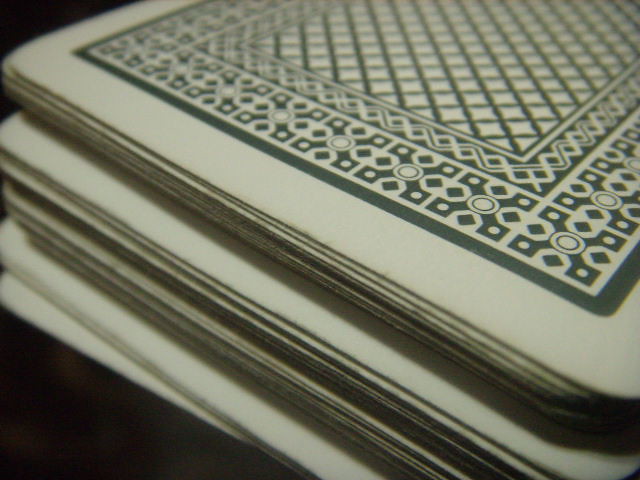The image features a neatly stacked deck of playing cards, arranged in a manner that suggests it is a complete set. The photograph is taken from a close-up angle, allowing for a detailed view of the card tops. Each card is predominantly white, adorned with a dark green, Moroccan-inspired checkered pattern. This intricate design is reminiscent of a mesh fence, adding a touch of elegance to the otherwise ordinary deck. Despite the zoomed-in perspective, which limits visibility of any suits or numbers on the cards, the uniformity and detailed pattern of the card backs are clearly discernible. The deck appears freshly opened, with all cards perfectly aligned, showcasing the distinctive and aesthetically pleasing design.